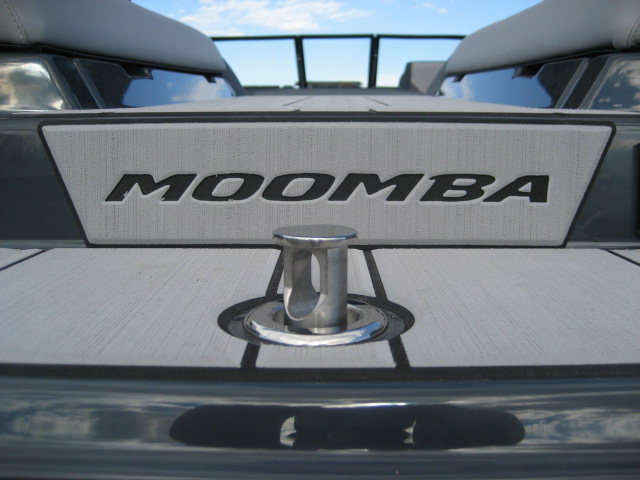The image depicts the rear section of a Moomba boat, captured closely on a sunny day with a clear blue sky and fluffy white clouds. The boat's light gray deck features darker gray trim along the sides and at the bottom center. Prominently displayed in the middle of the frame is the logo 'Moomba' in black writing, embossed on a white panel. Below the logo, there is a silver cylindrical object, possibly a tow bar or a tie-point for a rope. The glossy blue fiberglass elements of the boat reflect the vibrant sky, and white padding provides a comfortable seating area on either side of the flat deck. The image extends towards the front windshields, offering a view into the boat's interior seating area, further detailed with additional planking and trim.